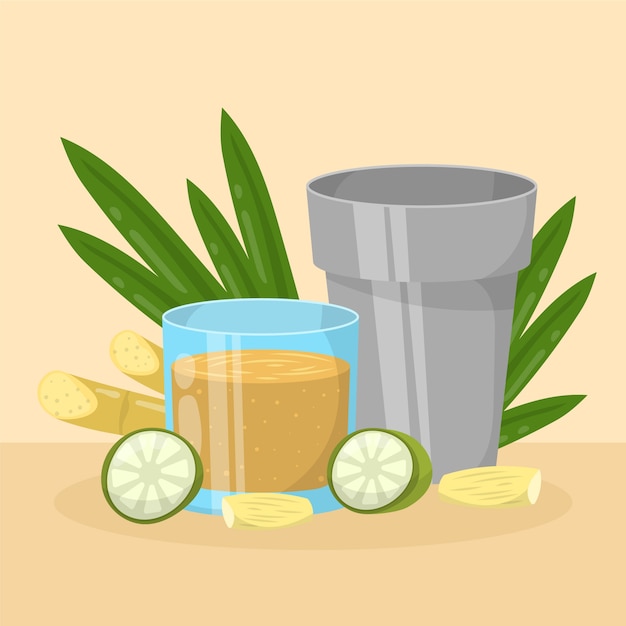This computer-generated graphic, set against a peach background, artfully arranges various elements into a pleasing composition. On the right, a purple plant pot with a distinct lip and graduated base showcases two medium green palm frond-style leaves elegantly fanning out on either side. Beside the pot, a turquoise glass filled with a thick, peanut butter-colored liquid stands prominently, accentuated by two lime halves placed on either side. Scattered near the glass are two tan almonds, adding a touch of organic texture. On the left, two sliced cylinders resembling cut baguette pieces are neatly positioned, their golden-brown hues balancing the scene. The combined elements create a visually compelling and harmonious still life.